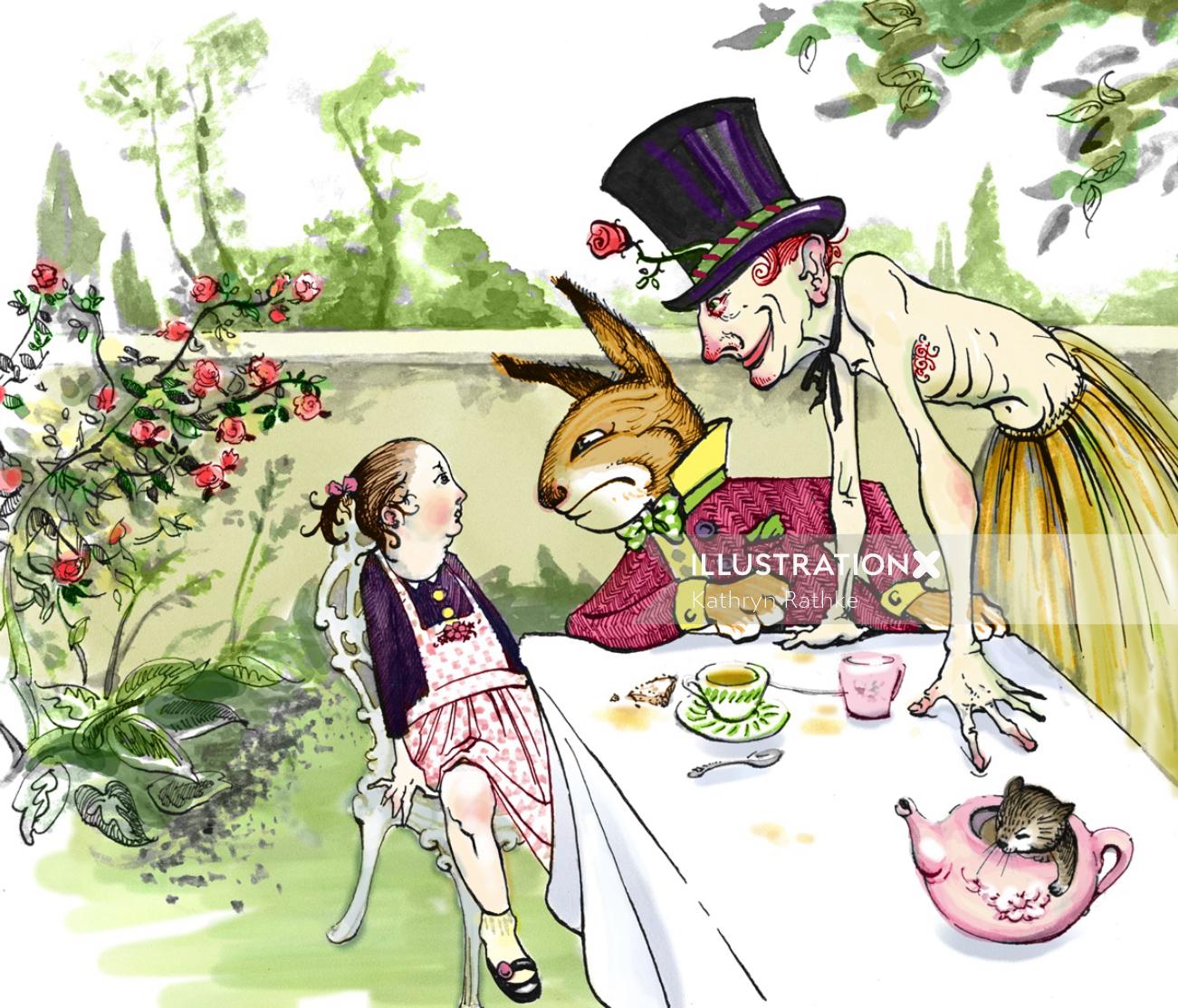This illustration by Kathy Rath offers a modern, abstract depiction of the classic "Alice in Wonderland" tea party. Alice is seated at the table, dressed in a red and white checkered dress over a black shirt. She leans back with a worried expression on her face as the Rabbit, clad in a purple shirt with gold cufflinks, a green bowtie, and a yellow collar, peers menacingly inches from her face. To her right, the exceedingly thin Mad Hatter sports an evil grin, a bright pink nose, a large purple hat adorned with a rose, and what appears to be a hula skirt. His fingers, unnaturally skinny and creepy, add to the scene's eerie atmosphere. The tea party setting includes a teacup, a tea container, and a spoon on the table, surrounded by few stylized plants and roses to the right, with the teacup being green and other containers in pink. The entire composition is both whimsical and unsettling, highlighting Rath's unique, modern take on this beloved story.